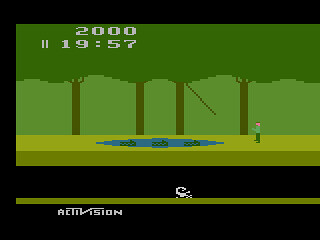A screenshot from a retro-style video game by Activision. The screen prominently displays the text "2000" and "1957," which might represent the player’s score or the in-game time. A character is shown on the right side of the screen, facing a section of water in front of them. Emerging from the water are three green, alligator-like heads, appearing to obstruct the character’s path. The objective seems to be navigating this obstacle, possibly to advance to the next level. The game's overall aesthetic is reminiscent of classic arcade games, featuring a black background that enhances its vintage appeal.